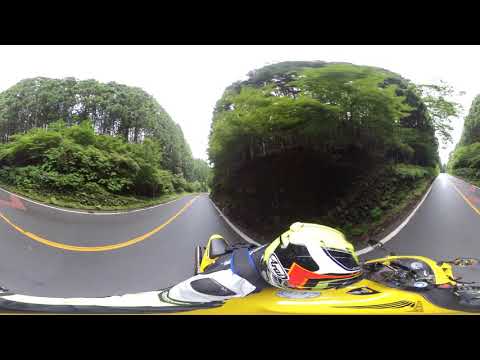The image is a heavily distorted double fisheye photograph presenting a surreal street scene. Dominating the lower part of the image is a bright yellow motorcycle, stretched and warped, with a figure in a white uniform and helmet riding it. The foreground is marked by shiny, wet asphalt with distinctive yellow divider lines that curve and snake across the frame, adding to the image's visual confusion. The street is flanked on both sides by lush, massive green trees, creating a verdant corridor. The sky appears hazy and overcast, contributing to the overall cloudy ambiance of the picture. Black horizontal bars frame the top and bottom of the image, enhancing the distorted and dreamlike quality of the scene. The unique lens effect makes the road appear to bend in unusual ways, further intensifying the sense of distorion and surrealism.